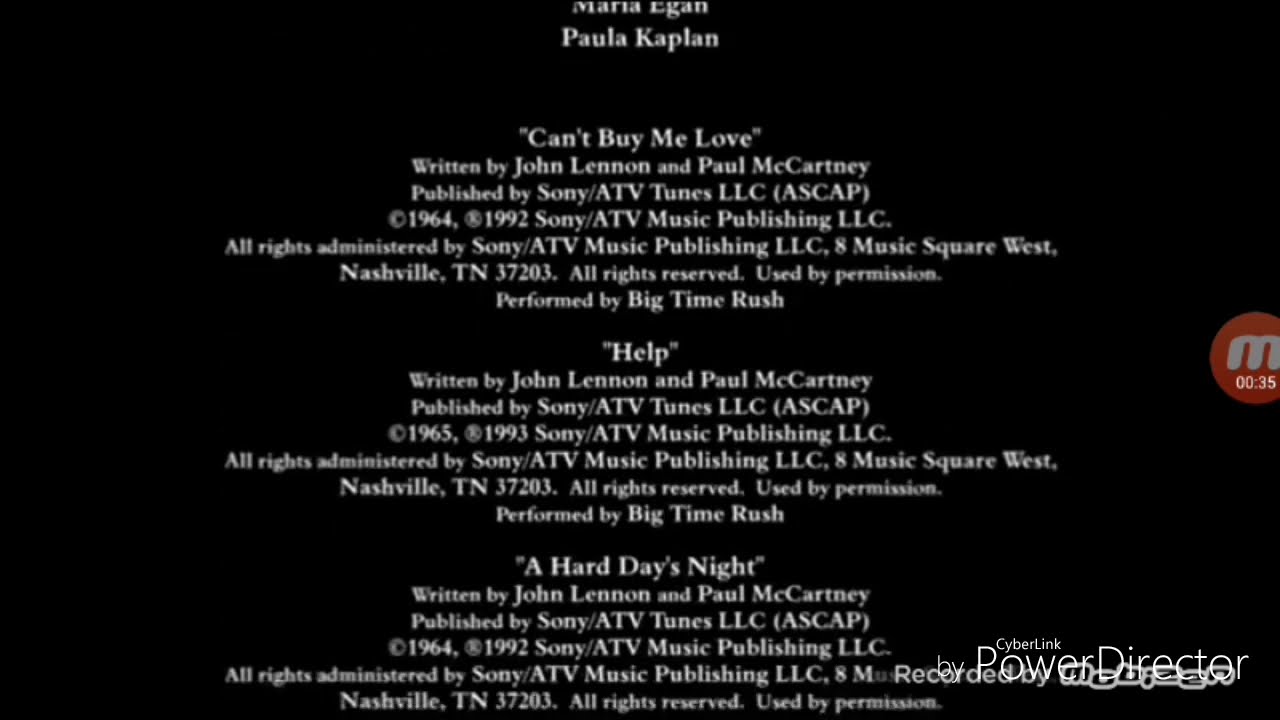The image depicts the end credits of what appears to be a movie, showcasing a monochrome layout with a black background and white text. It lists three iconic Beatles songs: "Can't Buy Me Love," "Help," and "A Hard Day's Night," all credited to John Lennon and Paul McCartney. Each song credit includes detailed publishing information and notes that they are performed by Big Time Rush. Additional names, Marla Egan and Paula Kaplan, are also mentioned in the credits. A red emblem featuring an "M" with the number 35, possibly a logo, is positioned on the right side, along with a mention of Cyberlink Power Director.